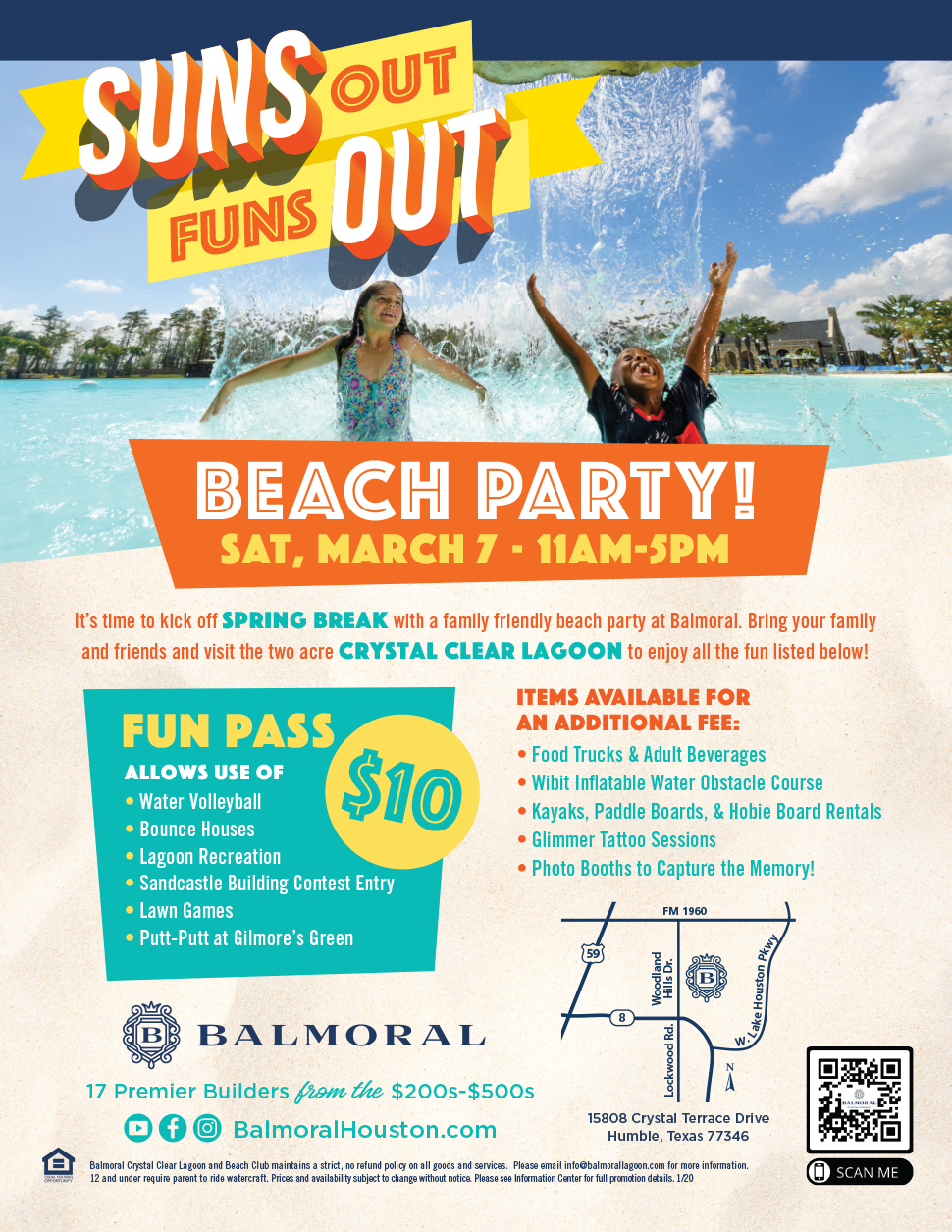The advertising flyer for the Balmoral Beach Party is vibrant and attention-grabbing, featuring the headline "Suns Out, Funs Out" in bold orange and white letters on a yellow ribbon, though it lacks an apostrophe for grammatical correctness. This catchy caption is superimposed over a joyful black-and-white image of children splashing and playing in a swimming pool. The event details are prominently displayed: "Beach Party, Saturday, March 7th, 11am to 5pm." 

The flyer invites families to kick off spring break at Balmoral, promising a host of activities at the stunning 2-acre Crystal Clear Lagoon. For $10, a Fun Pass grants access to water volleyball, bounce houses, lagoon recreation, sandcastle building, contest entries, lawn games, and putt-putt at Gilmore's Green. Additional attractions, available for an extra fee, include food trucks, adult beverages, inflatable water obstacle courses, kayaks, paddle boards, hobie board rentals, glimmer tattoo sessions, and photo booths to capture memories.

The flyer is designed in bright, beachy colors like yellow and turquoise, enhancing its festive appeal. A small map is included for directions, along with the website BalmoralHouston.com, and logos for Facebook, Instagram, and another unspecified social media platform. At the bottom right, a QR code with the prompt "scan me" provides more information. Mention is made of 17 premium builders with homes priced from the $200s to $500s, suggesting this is a planned community.